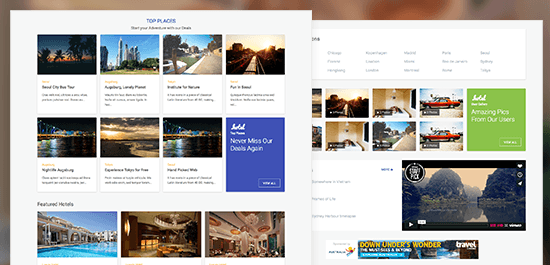The image showcases two adjacent web pages filled with vibrant visuals and travel-related content. The left page is titled "Top Places" at the top, featuring various captivating destination images such as beaches, buildings, and streets. The design is minimalistic with a gray-white background, adorned with pictures accompanied by brief descriptions. Towards the bottom left, there is a section labeled "Featured Hotels," displaying three images of different hotels. Above this, on the right side, there is a promotional button or ad that reads "Never Miss Our Deals Again."

The right page mirrors the visual richness of the left, with an emphasis on diverse imagery and content options at the top. It includes a green-highlighted section titled "Amazing Pics from Our Users," inviting viewers to explore user-generated photos. Lower on the page, there are advertisements for "Down Under's Wonder Travel" from the travel channel. Additionally, there's an embedded video that users can play, showing a preview image of a serene river flanked by majestic mountains, enhancing the travel-themed aesthetic of both pages.